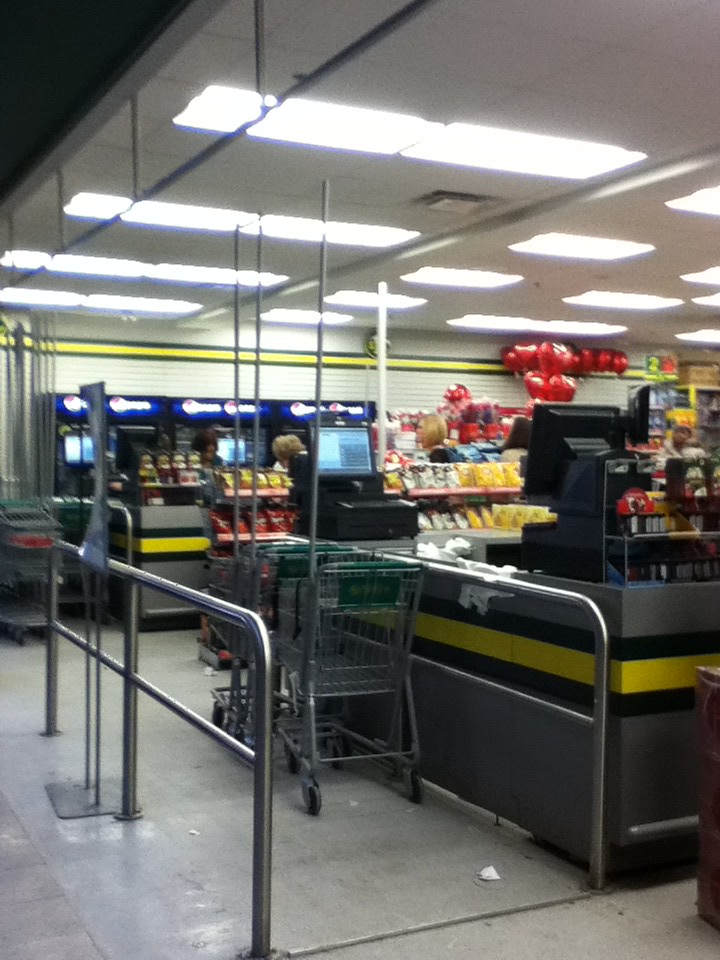The image depicts the interior of a slightly blurry grocery store or convenience store, likely photographed from the entrance at night. Dominating the scene is a metal corral filled with shopping carts, which have notable green handles and extend towards the ceiling with large poles. The ceiling above features traditional drop tiles illuminated by large, rectangular white fluorescent lights, providing ample light for the setting. A prominent yellow stripe runs along the top of the wall.

Towards the right side of the image, there are several checkout aisles, each with gray counters outlined in black and topped with disorganized papers or paper towels. Just beyond these, the scene includes vending machines and shelves stocked with snack bags, some prominently displaying chips. Red heart-shaped balloons float near the ceiling in the background, adding a touch of festivity.

Additionally, near the back of the store are a few older women and at least one African-American individual appearing to glance towards the camera. The floor, covered with gray linoleum, shows signs of casual disarray, such as scattered bits of trash. The overall scene conveys a sense of everyday activity and casual clutter within the store.